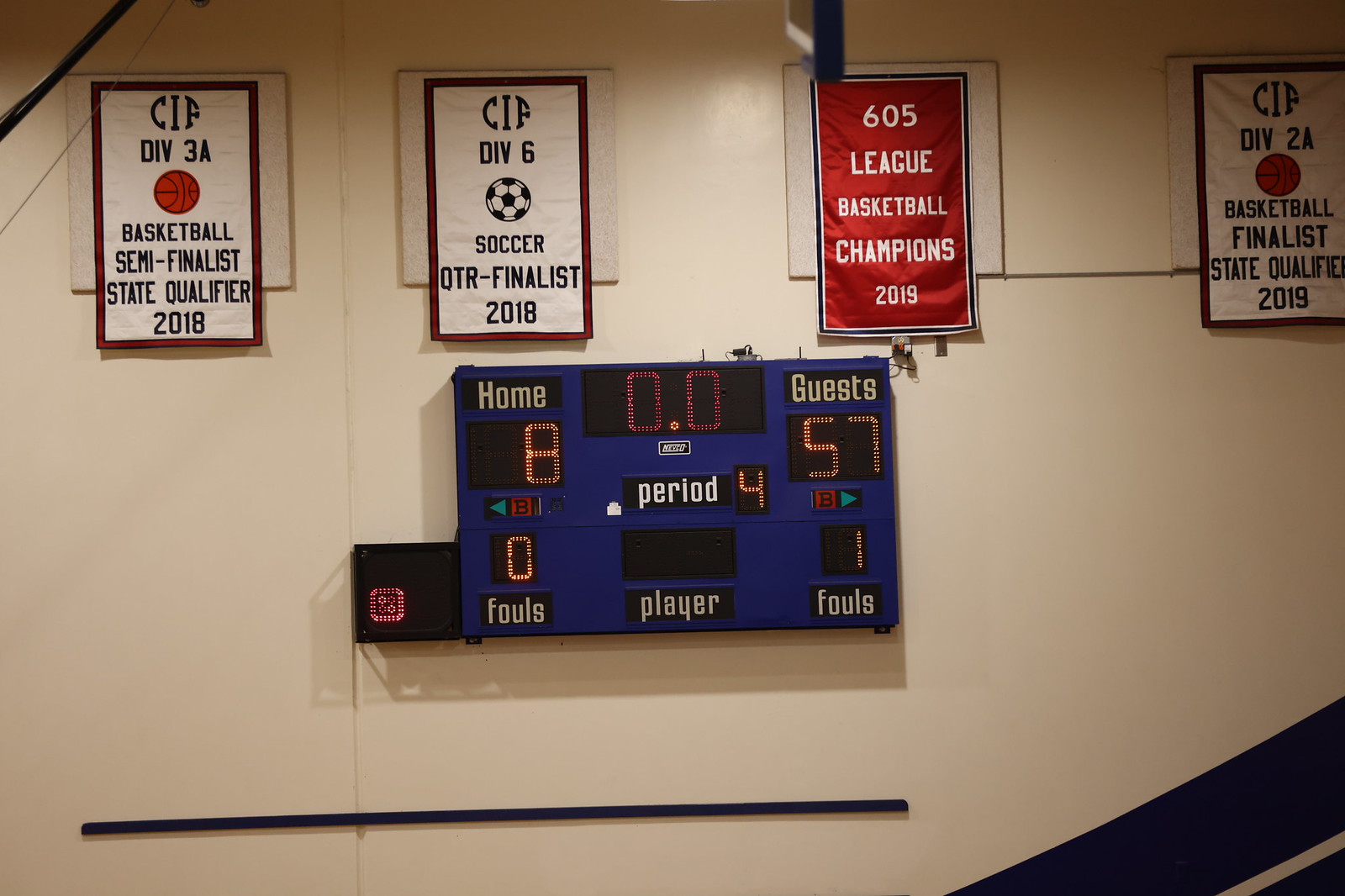The image depicts a gymnasium wall adorned with various sports banners and a digital scoreboard. From left to right, the first banner is white with a brown border and reads "CIF Division 3A Basketball Semi-Finalist State Qualifier 2018," featuring an orange basketball graphic. Next, a similar white banner with a black border shows "CIF Division 6 Soccer Quarter-Finalist 2018" with a soccer ball illustration. Adjacent to this is a red banner bordered in black and white, stating "605 League Basketball Champions 2019" in white lettering. The fourth banner on the right, also white with a brown border, is labeled "CIF Division 2A Basketball Finalist State Qualifier 2019" in black font. Below these banners, a dark blue electronic scoreboard displays "Home" with a score of 8 and "Guests" with a score of 57 in the fourth period, along with foul counts indicating zero for the home team and one for the guests, all set against a beige wall with a black streak running in the lower right corner.